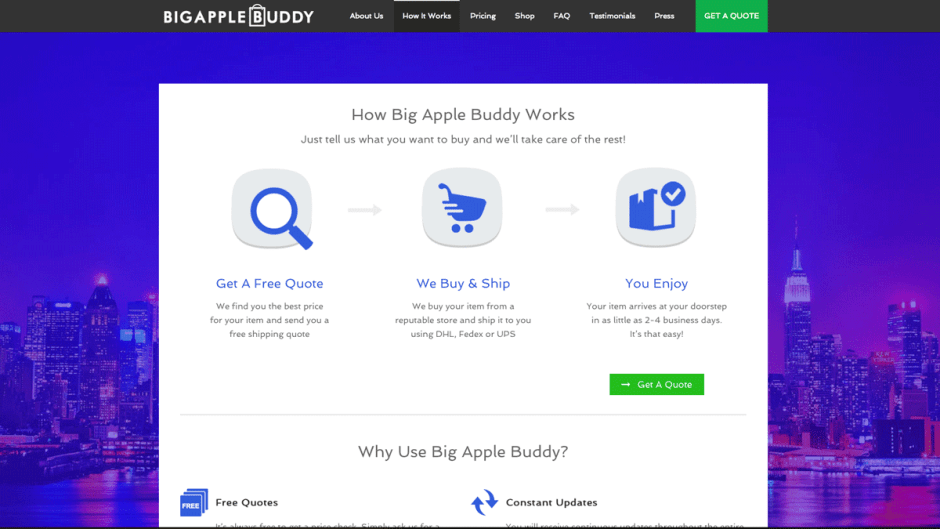This is a horizontally aligned rectangular image that exhibits an organized blend of textual and graphical information. The upper portion of the image is a black banner containing the brand name "Big Apple Buddy" in white capital letters, formatted to appear as one word. The "B" in "Buddy" is visually integrated with a small shopping bag icon, adding a distinctive touch. 

Following this, there is a series of menu options in white letters, spanning from the left of center to approximately halfway across the image: "About Us," "How It Works," "Dining," "Shop," "FAQ," "Testimonials," and "Press." 

A prominent feature on the right side of this black section is a green button with white capital letters reading "GET A QUOTE."

Beneath this is a large white rectangular area superimposed over a scenic city backdrop. The cityscape features a blue sky with various buildings peeking from either side, their reflections shimmering in the water below, bathed in a subtle pink glow. 

Centered within the white rectangle, bold text states, "How Big Apple Buddy Works," followed by a smaller, more detailed explanation: "Just tell us what you want to buy and we'll take care of the rest."

The explanation is divided into three sections:

1. The first part, "Get a Free Quote," features a magnifying glass icon within a white square, highlighted with blue text. Below, black text elaborates, "We find you the best price for your item and send you a free shipping quote."

2. The second part, "We Buy and Ship," includes an icon of a shopping cart within a white square and blue text. The accompanying description reads, "We buy your item from a reputable store and ship it to you using DHL, FedEx, or UPS."

3. The third part, "You Enjoy," is symbolized by an icon partially blue and partially white, with a prominent blue checkmark. The text states, "Your item arrives at your doorstep in as little as 2-4 business days. It’s that easy."

Below this, a green rectangular button with white lettering once again prompts viewers to "GET A QUOTE."

At the bottom of the page, the text highlights "Why Use Big Apple Buddy?" with two sections: "Free Quotes," accompanied by an icon on the left, and "Constant Updates," similarly paired with an icon to its left. 

The clean, organized layout effectively conveys the various aspects of Big Apple Buddy’s services and their unique selling propositions.